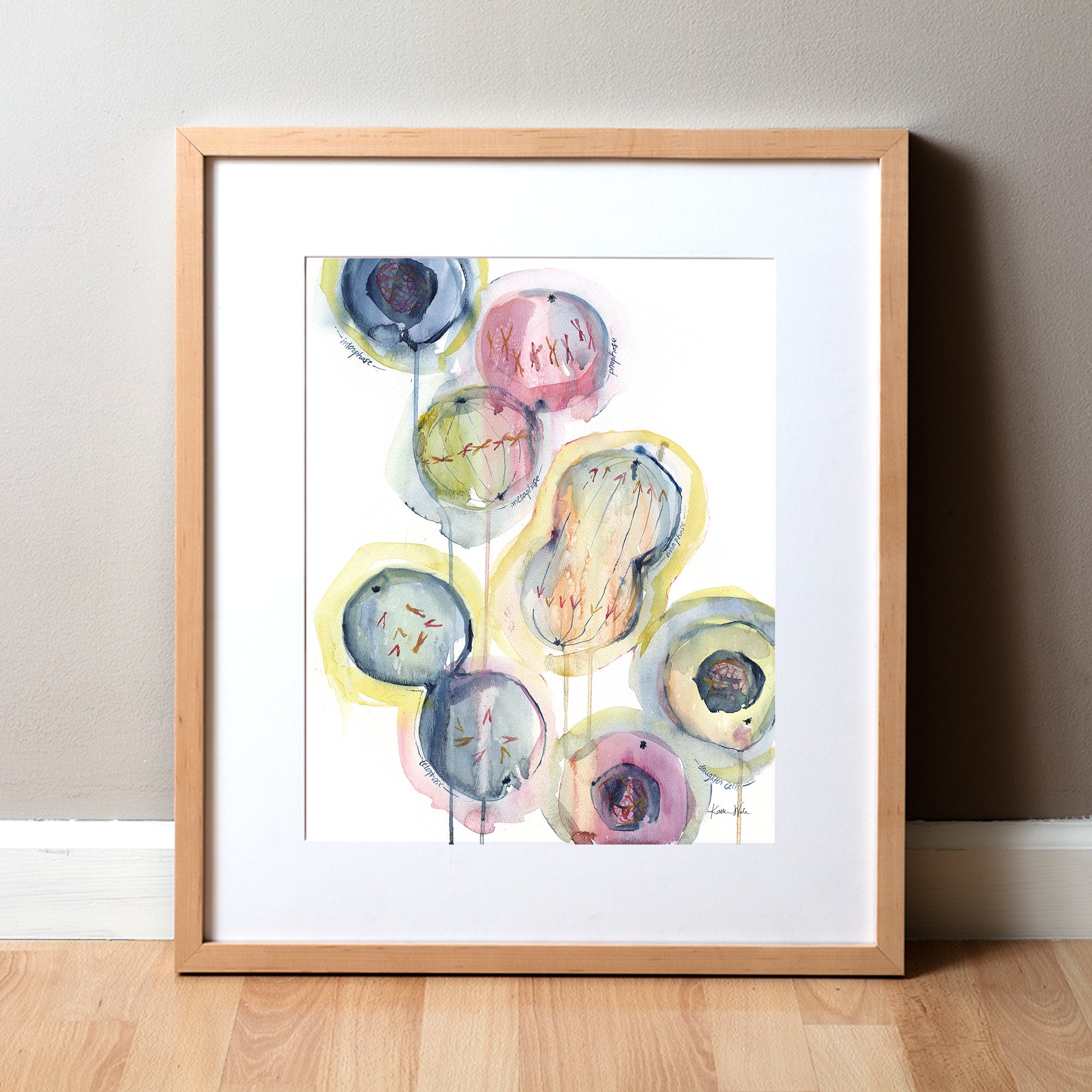This photograph appears to be taken from a seated position on the floor. It showcases a framed picture leaning against the wall. The floor features light blonde hardwood, and the wall is a subtle stone gray with a white baseboard at the bottom. The frame of the picture is made of light, unfinished wood, and it contains a thick, off-white mat. The artwork within the frame is a colorful and sketchy watercolor painting. It depicts a collection of pastel-hued objects resembling Chinese lanterns or balloons in various colors, including pink, blue, green, and yellow. There are nine of these objects in total, all seemingly floating upward, each anchored by distinct dark strings trailing downward. The design of the balloons includes intricate patterns with different shapes and concentric circles within them, adding to the whimsical and vibrant nature of the piece.